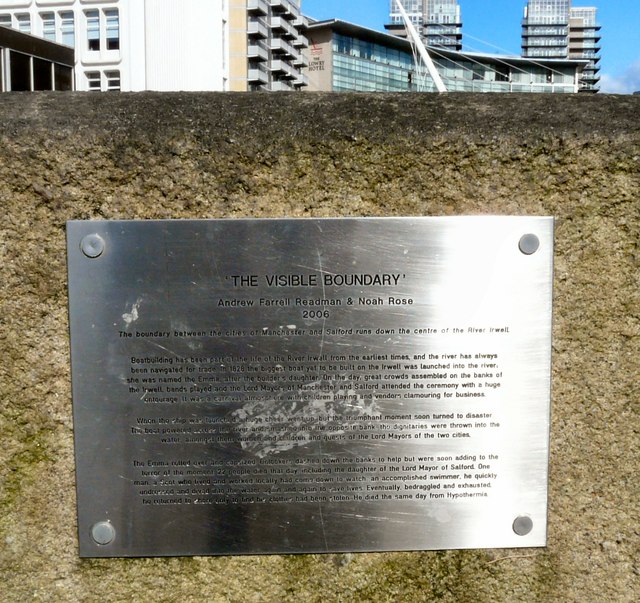The image showcases a silver metal plaque mounted on a moss-covered stone wall. This plaque takes up most of the photo, with the top quarter revealing a blue sky and looming buildings in the background, including a curved structure, likely the Lowry Hotel, and a taller nearby building. The plaque is engraved with dark-colored text, reading "The Visible Boundary," followed by the names "Andrew Farrell, Redmond, and Noah Rose, 2006." Below this header, the first line states, "The boundary between the cities of Manchester and Salford runs down the center of the River Irwell." The remaining three paragraphs of text are difficult to decipher due to the plaque's weathered condition and the small font size.